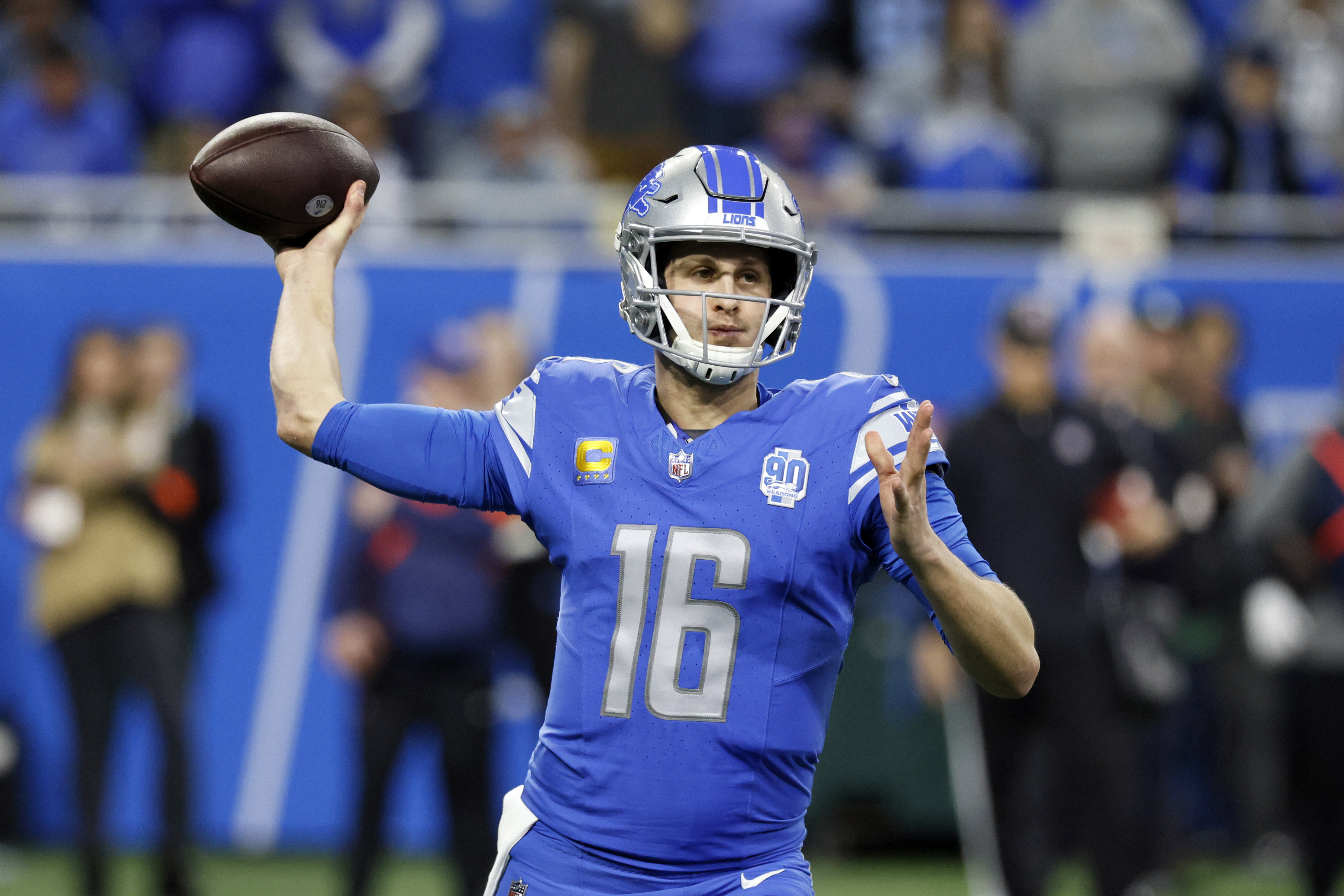The photograph captures NFL player Jared Goff in the midst of throwing a football during a game. Dressed in the Detroit Lions' blue jersey with the number 16 in silver, Goff is poised with his left hand extended in front and his right arm cocked back, clutching the football. His jersey features distinctive silver stripes on the shoulders, and beneath it, he wears a longer-sleeved blue shirt reaching his elbows. Prominently displayed on the upper left corner of his jersey is a gold captain's "C," while the upper right corner bears a decal with the number 90, and centered between them is the NFL logo. Goff's helmet is silver with three blue stripes running down the middle and "Lions" visible just above the visor. He maintains a focused and serious expression as he prepares to throw. In the background, blurred to keep the focus on Goff, are fans in the stands and people appearing in blue attire, reflecting the team’s colors. The overall scene suggests action within a live football game, putting emphasis on Goff's readiness to make a play.